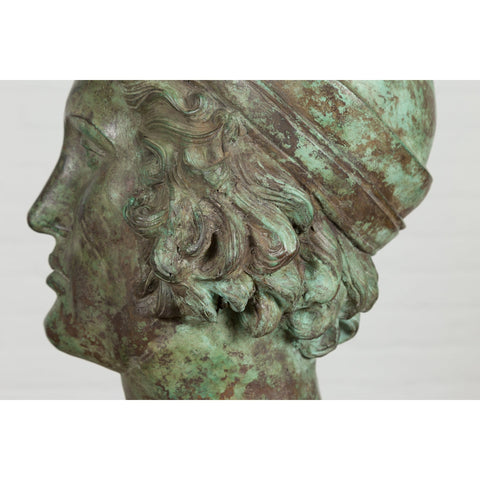This close-up photograph captures the aged and weathered head of a rusted statue, likely made of copper. The head, facing towards the left, is cropped at the top just above the forehead, revealing only the side profile. The statue has short, curly, or wavy hair tightly wound and is adorned with a multi-tiered snow cap showing significant green oxidation, typical of aged copper. The facial features include a prominent left eye, a long nose, and small lips, giving it a blank, indifferent expression. The chin juts outward slightly. The neck is partially visible, adorned with green moss-like oxidation spots, contrasting with the dominant dark brown rusted areas, especially concentrated around the hair and the hat. The overall color palette combines hints of green oxidation and brown rust, signifying its age and deterioration. The background against which the statue is set is a neutral beige or white, allowing the details of the statue's weathered surface to stand out prominently.